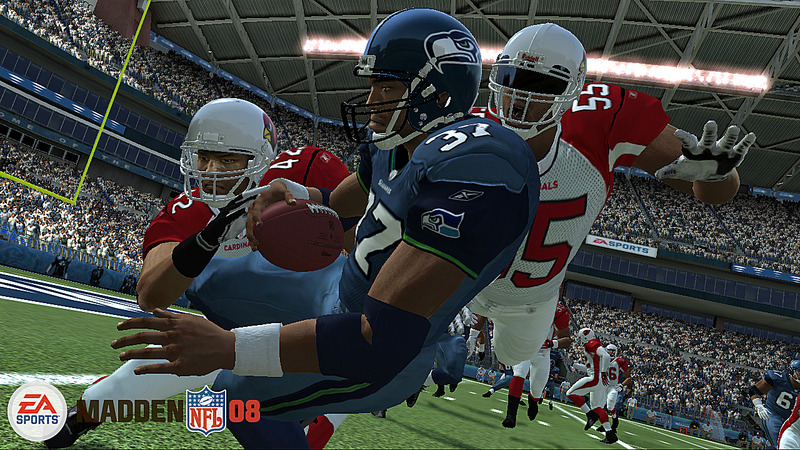This screenshot from the EA Sports video game Madden NFL 08 captures an intense moment between the Seattle Seahawks and the Arizona Cardinals. In this dramatic scene, a Seahawks running back, identified by his blue jersey with the number 37, is captured trying to evade a tackle from two Cardinals defenders dressed in red and white jerseys. The action takes place on a well-detailed, green field with white yard lines, emphasizing that the play is near the end zone, as the goal post frame is visible. The image also showcases a massive, fully packed domed stadium with thousands of fans dressed in white shirts, energetically cheering from the stands. The iconic EA Sports logo and the game's title, featuring black "Madden" text with the NFL logo and the red "08," are prominently displayed at the bottom.